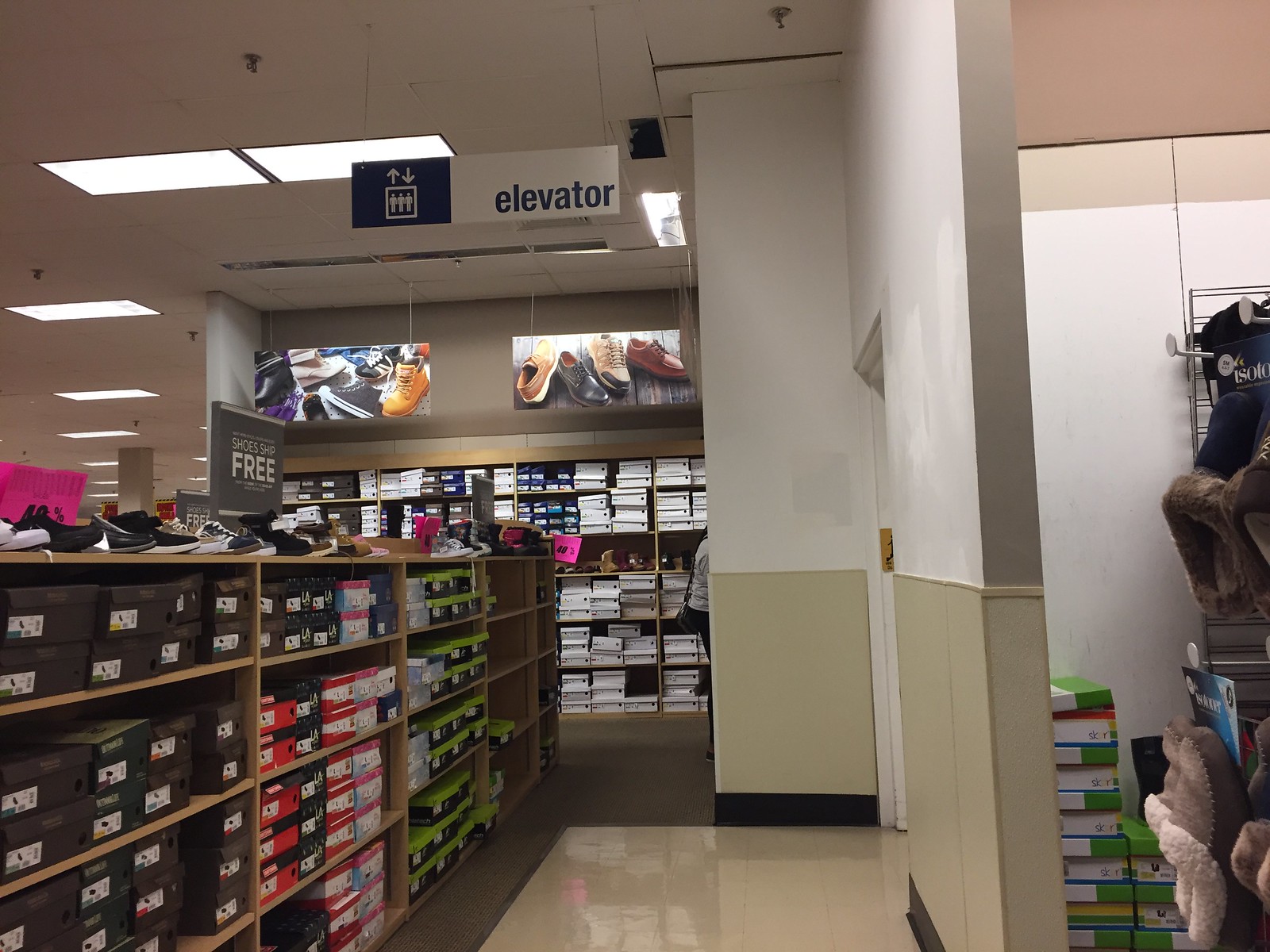The image captures the interior of a shoe store, showcasing a spacious layout with a mix of shiny light brown flooring and brown carpet. Dominating the scene are extensive shelves laden with shoe boxes in an array of colors, such as black, green, red, and blue, indicating different brands and sizes. The left side of the image prominently features tall, segmented shelving units filled to capacity with these boxes, topped with a variety of shoes displayed at a diagonal angle. A large promotional sign atop these shelves highlights a "Buy One, Get One Free" deal, with the word "FREE" prominently visible. 

In the background, a wall adorned with large rectangular images of shoes and boots adds visual interest and marketing appeal. Beneath these images, more shelves are stacked with additional shoe boxes. To the right, another segment of the store appears to store shoes in what resembles a closet space. Near the top of the image, recessed rectangular lighting fixtures illuminate the scene evenly. 

Hanging from the ceiling at the center of the image is a sign indicating the presence of an elevator, depicted with stick figures and arrows showing the directions up and down, suggesting its location nearby and its capacity for four people. Adding to the detailed environment, subtle signage and additional shoes can be seen scattered throughout the store, enhancing the thematic consistency of a well-organized and fully stocked retail shoe department.